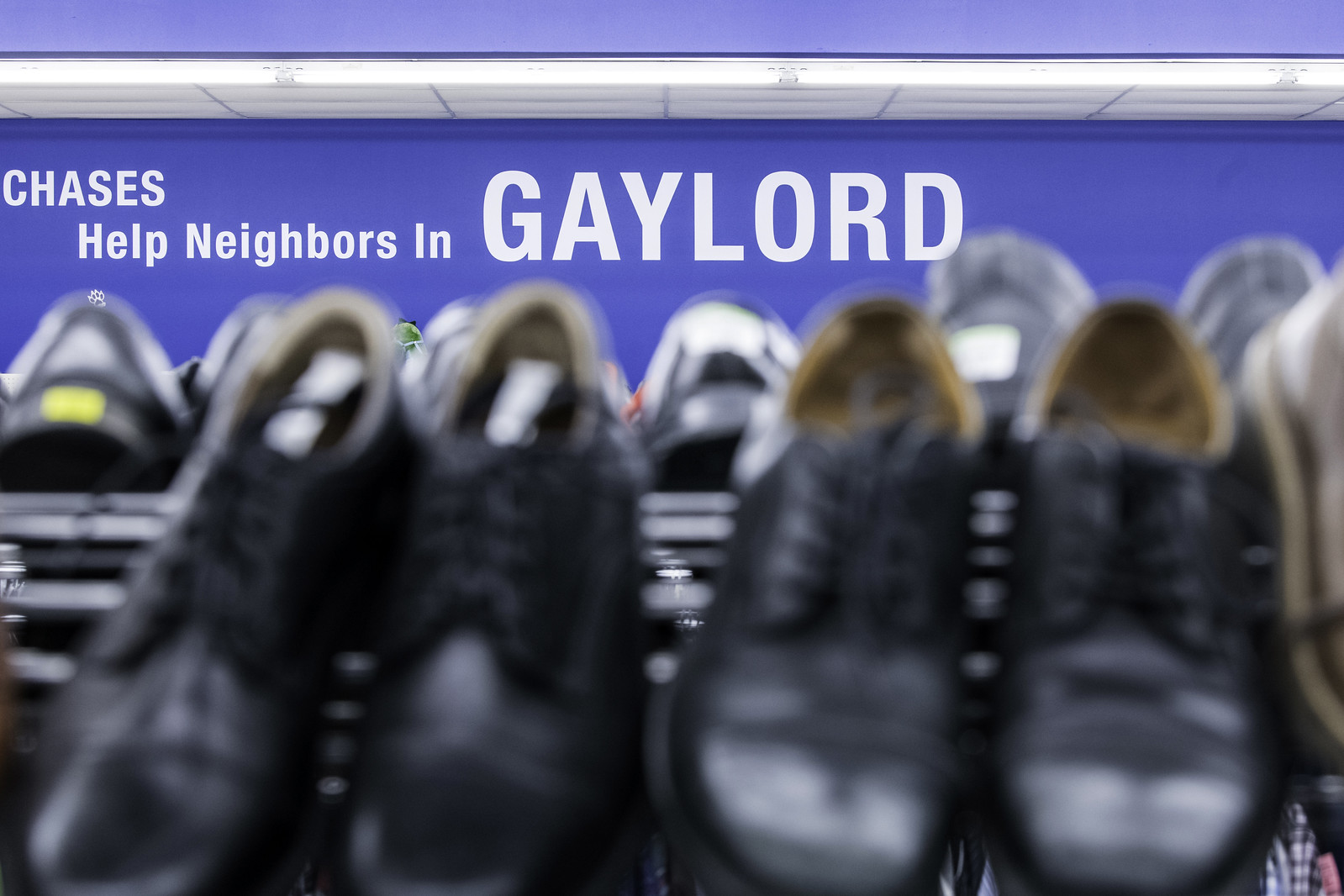The image portrays what appears to be a shoe store interior, characterized by a blue wall with white accents and text that reads, "Chases, help neighbors in Gaylord." The foreground features pairs of black shoes displayed on angled shelves, indicating they are possibly for sale. The background is filled with more shoes, although they are blurrier and in darker hues, similarly arranged on angled shelves. The overall scene suggests a retail environment, yet the mentioned text hints at a potential community support initiative, such as a shoe donation program. The visual cues, including the organized shelves and the signage, strongly imply a commercial setting, though the store's exact purpose remains partly ambiguous.